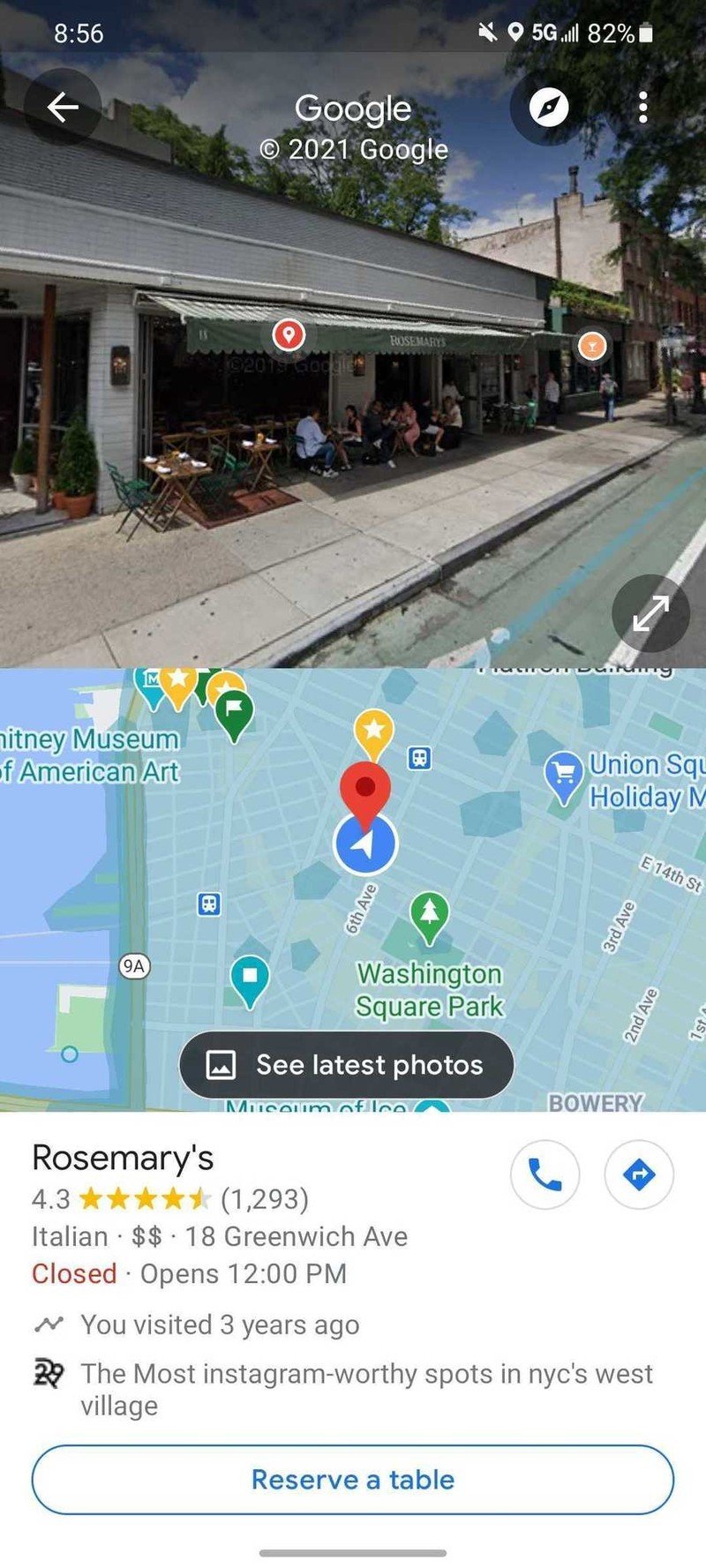The screenshot captures a moment at 8:56 AM, as indicated by the time displayed at the top left. To the top right, icons for image, location, 5G connectivity, signal strength, and battery life indicate an 82% battery charge. A back key is visible in the top left corner, and at the top center, the screen is labeled with "Google" and the copyright note "2021 Google."

The main content displays a view of some trees and a building in the background, which appears to be a restaurant with outdoor seating. Below this image is a map highlighting several key locations, including Union Square, Washington Square Park, 3rd Avenue, 2nd Avenue, and 6th Avenue. Additionally, a point of interest, Rosemary, is noted on the map with a rating of 4.3 stars based on 1,293 reviews.